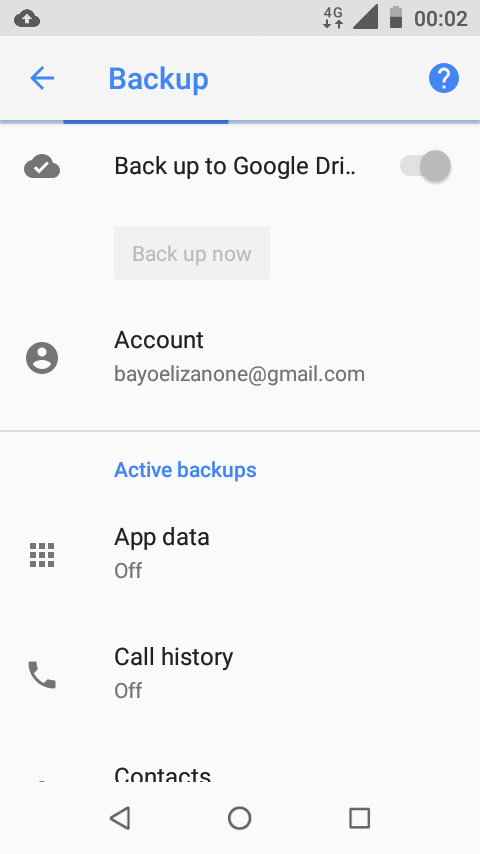This image is a screenshot of a smartphone's settings screen, specifically focused on the backup settings. The background is a standard gray, typical for settings screens, with various options available for toggling. 

At the top, the primary option is "Backup to Google Drive," which has a toggle switch currently set to off. Directly below this option, there is a grayed-out button labeled "Back up now." 

The next section is titled "Account," displaying the user's email address. Below this, separated by a gray divider line, is the "Active backups" section, highlighted in blue for emphasis. Here, the status of various backup categories is listed: "App data" is off, "Call history" is off, and "Contacts" is cut off, rendering the rest unreadable.

At the very bottom of the screenshot, the typical navigation icons of a Google phone are visible. In the center is a circle, serving as the home button. To the left is a left-facing triangle, commonly used for navigation, and to the right is a square, typically functioning as the app drawer button. The overall color scheme features black text, with the main title "Backup" and the subtitle "Active backups" in blue for clear distinction.